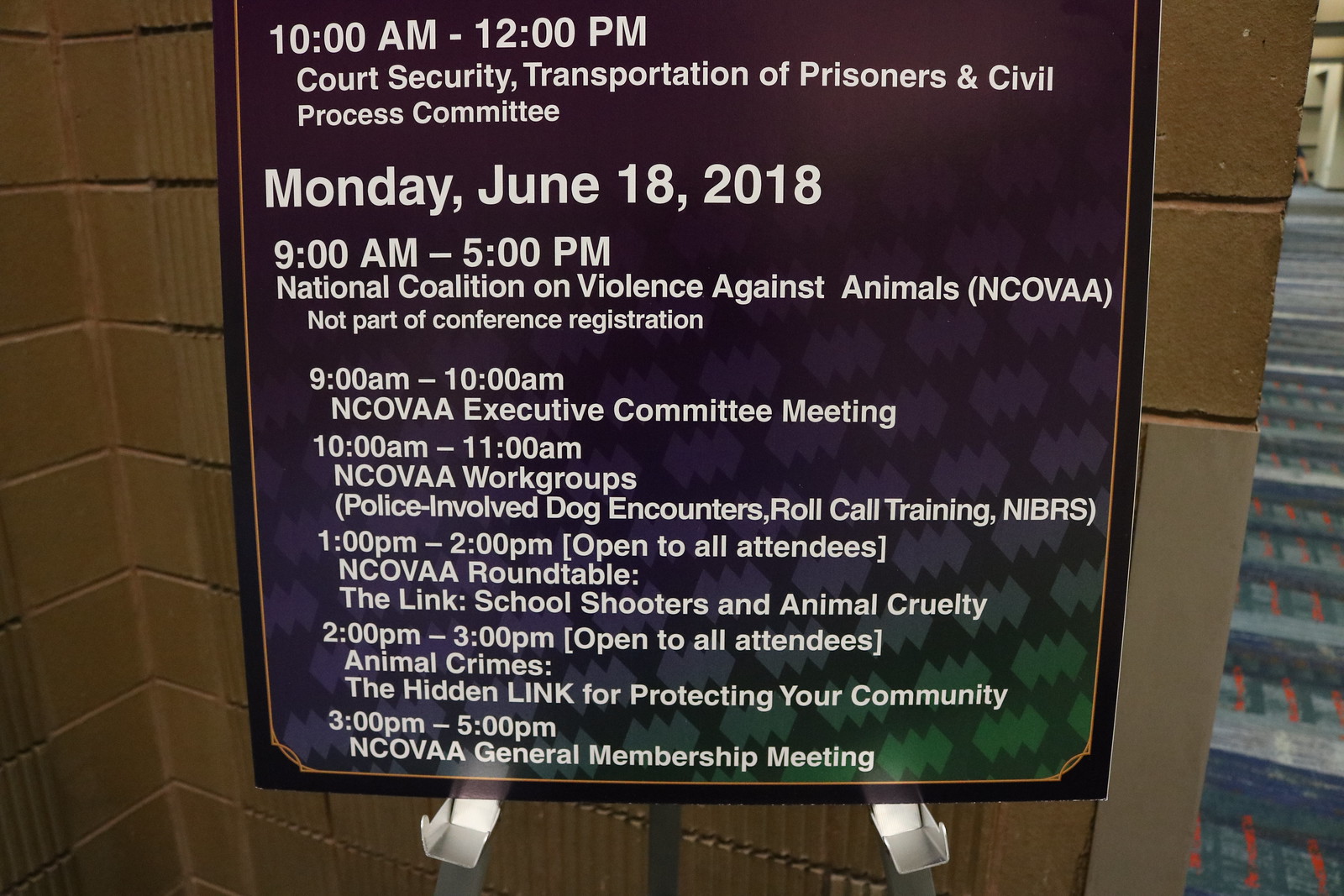The image depicts a detailed sign on a metal easel, set against a partitioned cinder block wall with a brick pattern, accompanied by carpeting in blue, red, and green stripes. The sign features a dark background with an ornate gold border and white text, describing the schedule and details for an event taking place on Monday, June 18, 2018. 

The agenda includes: 
- 10 a.m. to 12 p.m.: Court Security Transportation of Prisoners and Civil Process Committee.
- 9 a.m. to 5 p.m.: National Coalition on Violence Against Animals (NCOVAA) sessions, which are not part of conference registration.

Specific sessions for NCOVAA are:
- 9 a.m. to 10 a.m.: NCOVAA Executive Committee Meeting.
- 10 a.m. to 11 a.m.: NCOVAA Workgroups covering Police Involved Dog Encounters, Roll Call Training, and NIBRS.
- 1 p.m. to 2 p.m.: NCOVAA Roundtable on The Link, Animal Shooters, and Animal Cruelty, open to all attendees.
- 2 p.m. to 3 p.m.: A discussion on Animal Crimes and The Hidden Legacy, also open to all attendees.
- 3 p.m. to 5 p.m.: NCOVAA General Membership Meeting.

The sign effectively communicates the structured timeline and topics to be covered, providing clear guidance for attendees.